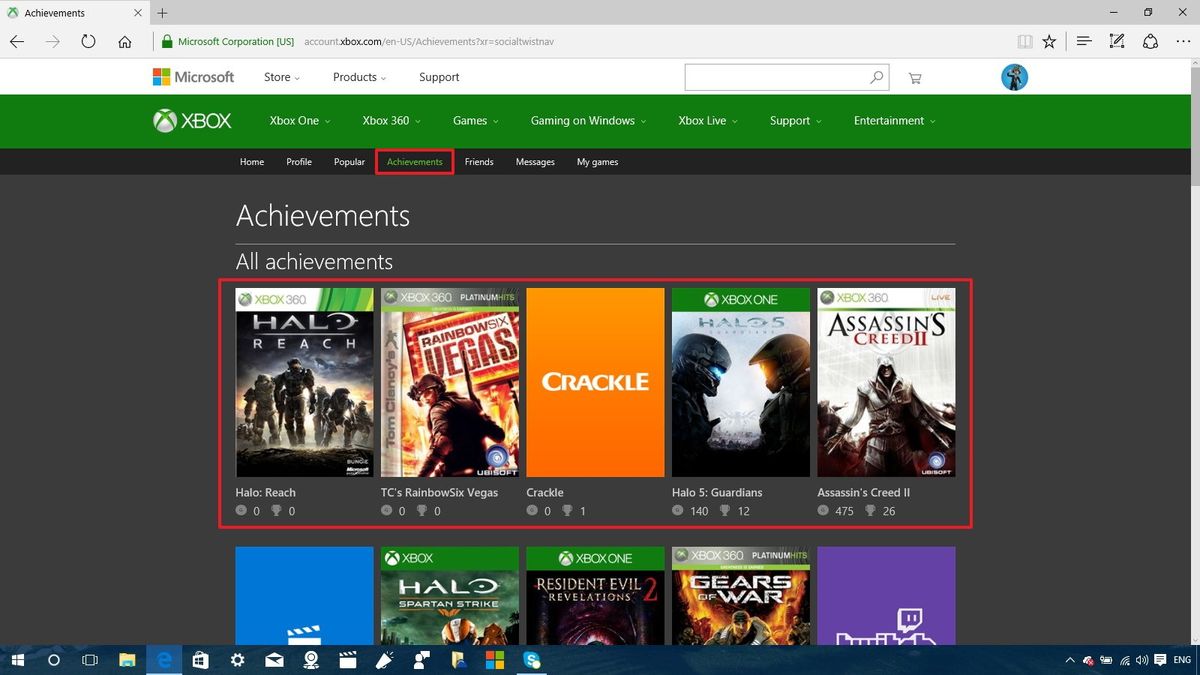The screenshot shows a webpage titled "Achievements," part of the official Microsoft Xbox domain (accountxbox.com), indicating a focus on Xbox gaming accomplishments. At the top of the page, within a red rectangular banner, the word "Achievements" is prominently displayed. 

The image features a list of Xbox 360 game achievements: "Halo Reach," "Rainbow Six Vegas," "Crackle" in an orange box, and another "Halo" game showing characters facing off. Other achievements illustrated include "Assassin's Creed 2," a blue icon with a white clapperboard, another "Halo" title named "Spartan Stride," "Resident Evil," "Gears of War," and a possible Twitch-related achievement. The visual arrangement emphasizes the top row, underscoring the achievements in a tidy, descriptive manner.